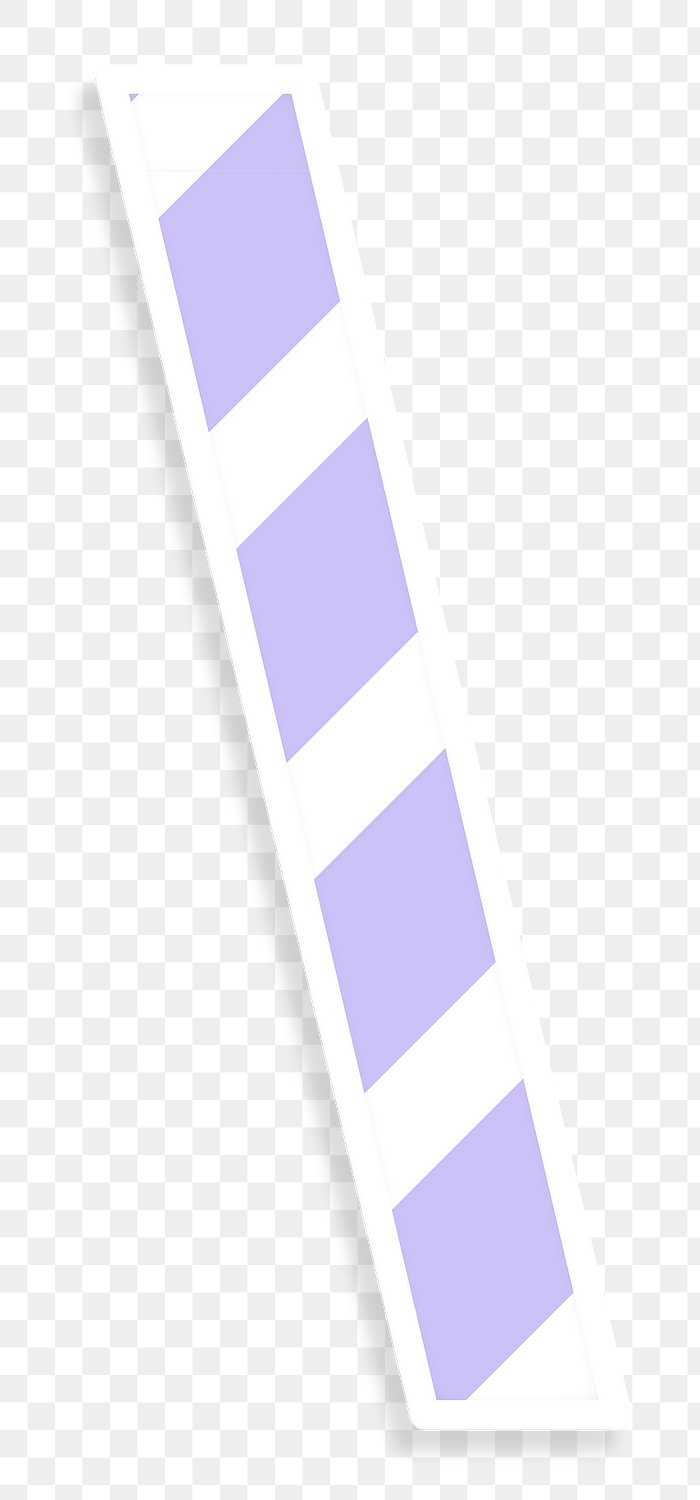This image features a long, skinny rhombus resting on a light gray and white checkerboard background. The rhombus itself is white, and within it, a repeating pattern of shapes is arranged in a linear sequence from top to bottom. Starting the sequence is a white triangle, followed by a purple diamond, then a white rhombus, another purple diamond, another white rhombus, a third purple diamond, yet another white rhombus, a fourth purple diamond, and finishing with a white triangle. The colors are pastel-ish, and the image appears to be computer-generated. The overall effect is of a meticulously arranged, elongated white strip adorned with alternating purple diamonds and white shapes, set against a soft checkered backdrop.